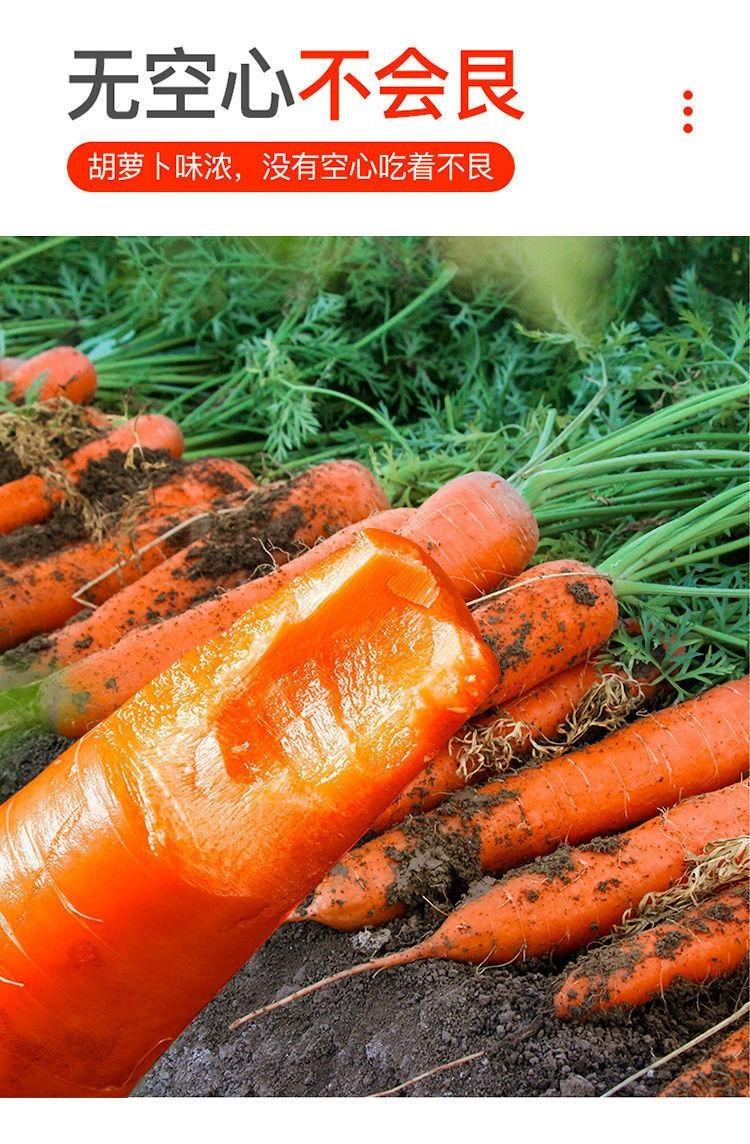This image features a detailed photograph of a pile of carrots freshly pulled from the ground, with their green tops still attached and covered in rich, black dirt. The carrots are angled from the lower left to the upper right of the picture, and prominently in the foreground, one carrot appears to be either broken or bitten off, revealing its moist interior. The photograph is framed with a white border, and the top quarter of the image is a white background hosting text in Asian characters, likely Chinese. The text comprises three grey characters followed by three orange characters. Below this text is an elongated, rounded orange text box containing additional white Asian script. To the right of this text box are three orange dots indicating a drop-down menu. This detailed composition suggests the photograph may have been taken from a website, capturing both the earthy, natural state of the carrots and the structured, informative layout of the digital interface.